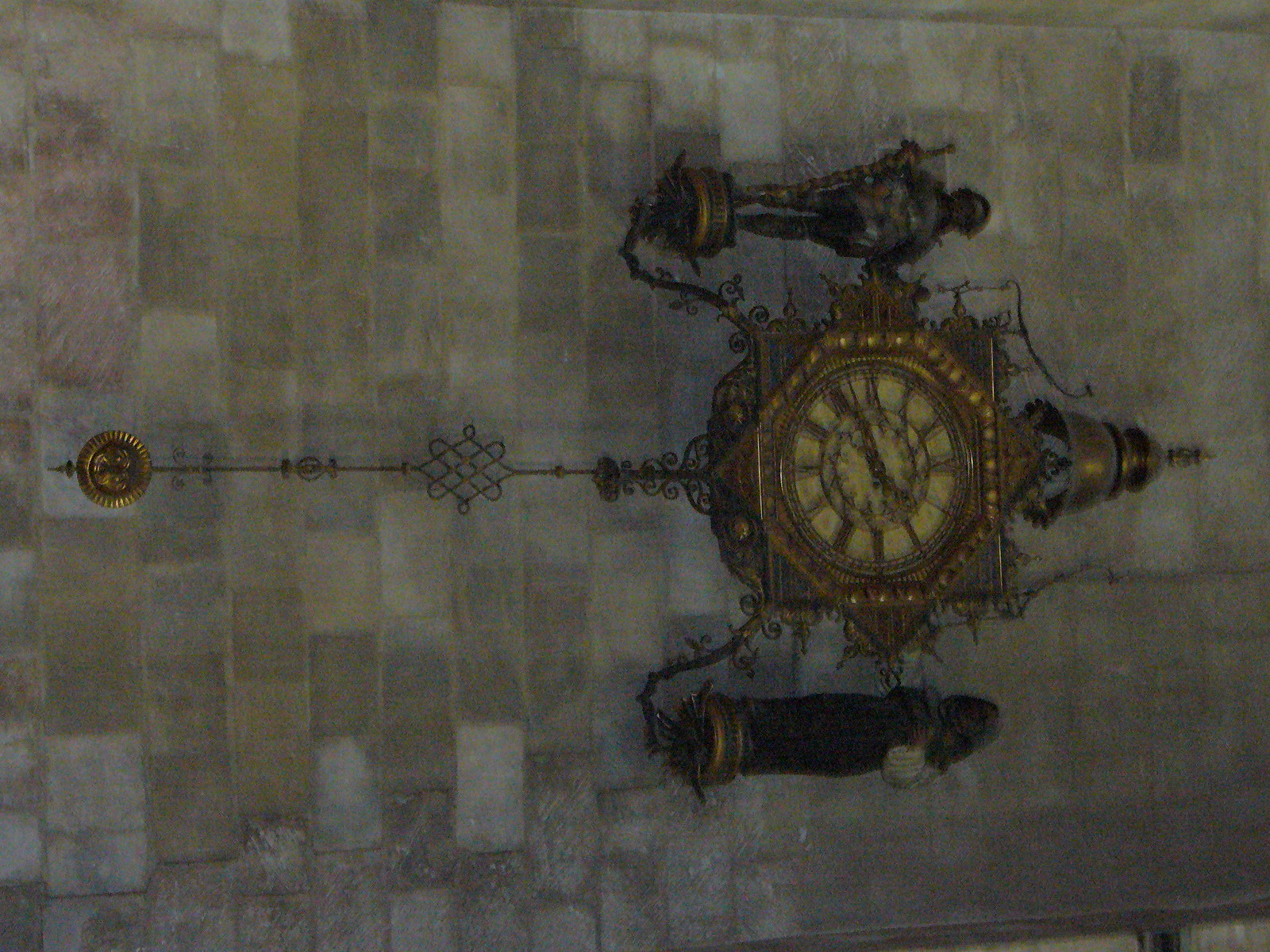The image showcases a digital rendering of a steampunk-style clock set against a textured light gray brick wall with variations in the brick tones. The clock, which has an old-fashioned aesthetic, features a square central face surrounded by a septagon-shaped golden frame. The intricate design includes a long, skinny pendulum hanging vertically to the left, ending in a circular gold disk. Adding to its ornate nature, the clock has two distinct statues on either side: the left figure resembles a soldier seated on a small platform with a curved arm extending to the clock, while the right figure appears to be a person in a dark cloak with a white arm, similarly positioned. Positioned atop the clock is a cylindrical, tapered bell with a pointed top, enhancing its elaborate design.